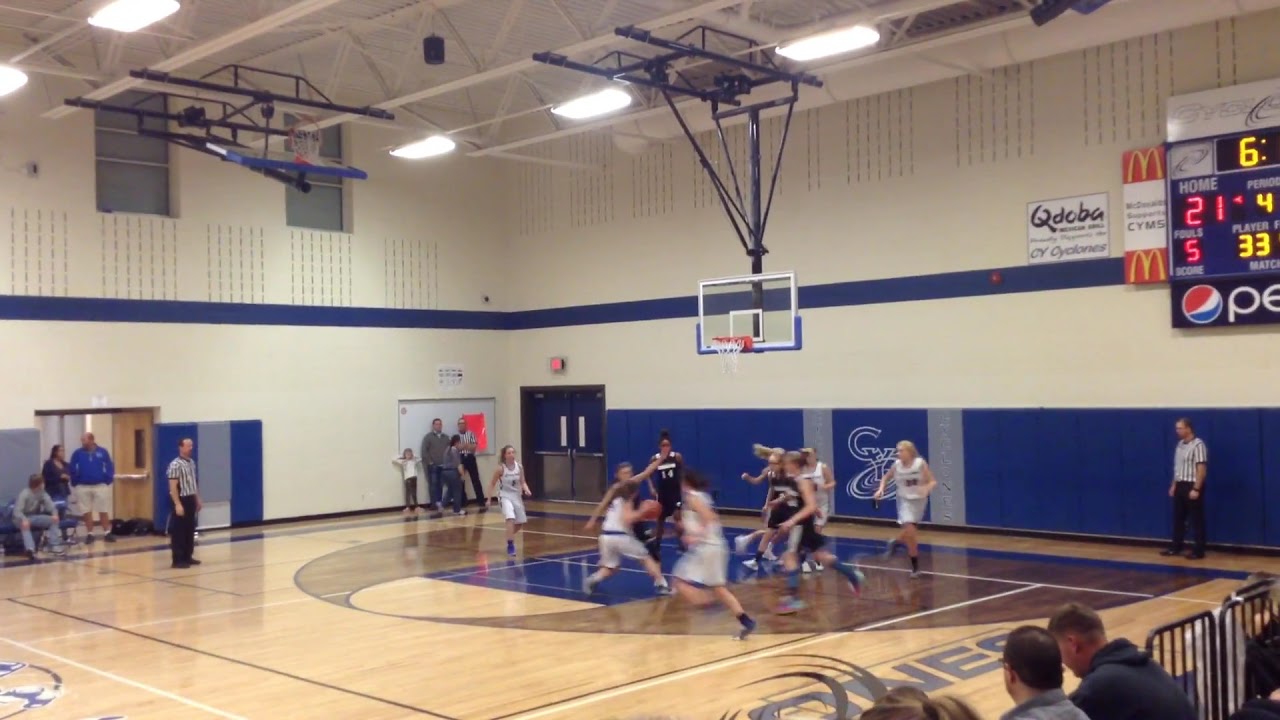In this indoor gymnasium setting, the photographic image captures an intense girls' high school basketball game in progress. The hardwood court, bordered in blue, features two teams: one dressed in white uniforms, the other in black. A player in white, holding the ball up in her arms, is closely guarded by a player in black. On the left side of the image, a referee intently watches the action, while another referee is positioned on the right. The audience's heads are visible to the bottom right, with more spectators lining the wall and standing in doorways. The walls of the gym are painted blue and white, and the scene is lit by fluorescent lights. Prominent on the court is a partial logo or lettering showing “N-E-S.” In the top right corner, a scoreboard displays the numbers 21, 6, 4, 33, and 5, beneath which is a “Pepsi” sign, partially visible as "P-E." Nearby, a McDonald's advertisement shows a large “M.” A basketball hoop hangs from the ceiling, completing the lively and detailed depiction of the game.